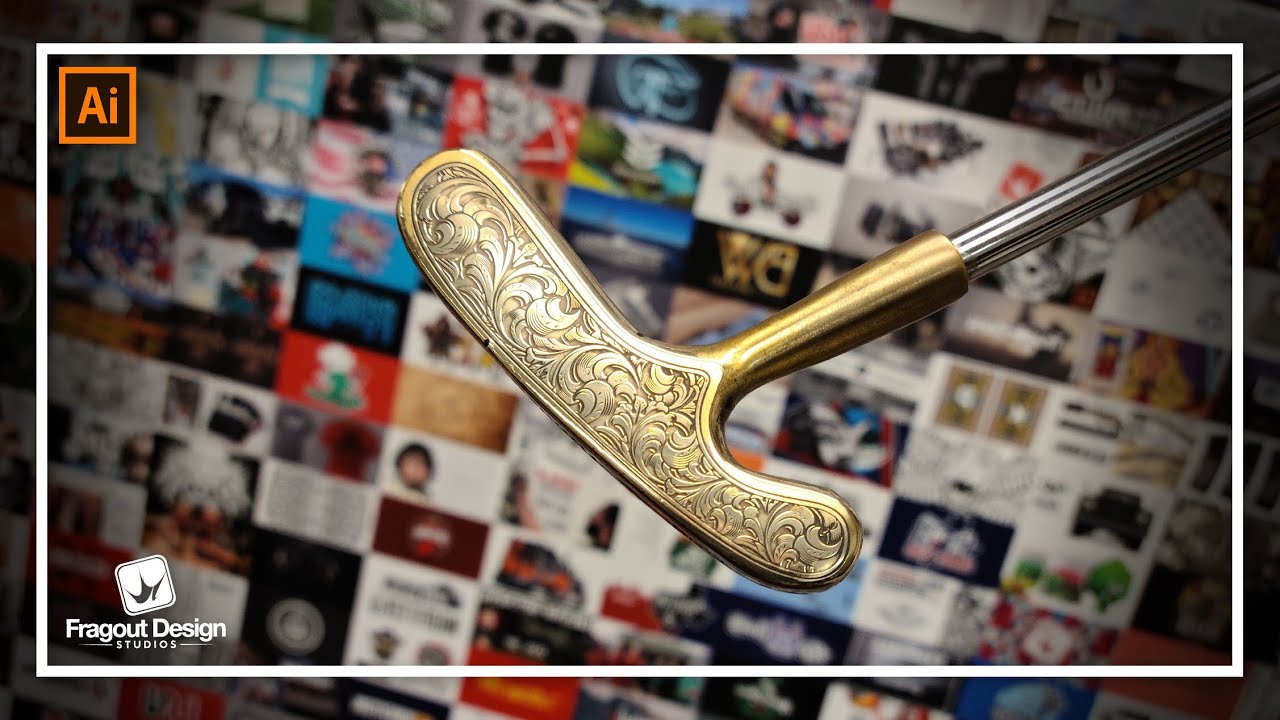This is a professionally produced photograph showcasing a beautifully designed putter, likely created using Adobe Illustrator as indicated by the orange "AI" logo in the top left corner. The photograph prominently features the putter emerging from the right-hand side, focusing on the intricate details of its design. The putter has a silver shaft leading to a bronze and gold head, adorned with elegant floral and feathery engravings which reflect exceptional craftsmanship. The handle appears untouched and pristine. In the bottom left corner, the image credits Frag Out Design Studios, denoted by their logo of a white crown within a square, and labeled text. The photo is framed by a white border, and the blurred background showcases an array of rectangular images, further highlighting the sophisticated look of the putter.